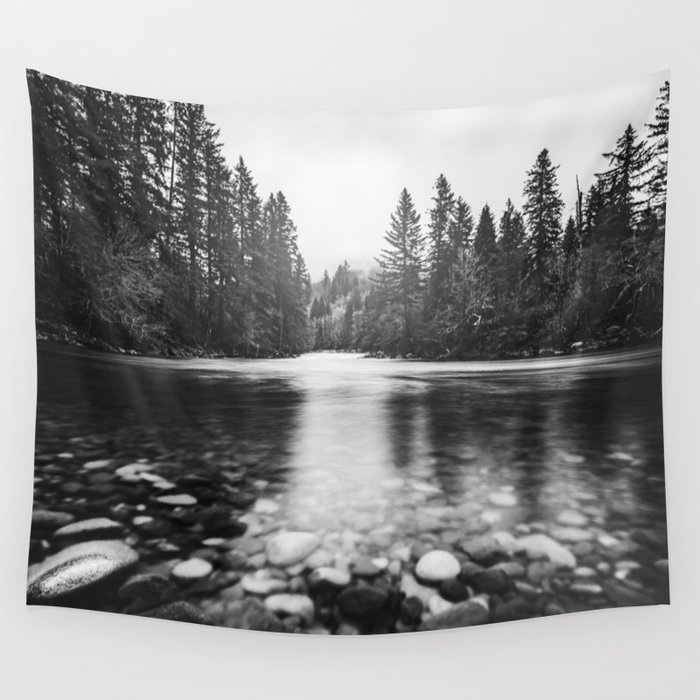This black-and-white image, possibly printed on cloth or used as a pillow cover, depicts a serene lake scene. The lake's surface is smooth and clear, reflecting the sunlight in a bright, white sheen that cuts across the water. In the foreground, there's a collection of round, worn pebbles and smooth rocks, their light coloration contrasting against the dark water. The background features a dense forest of tall pine and evergreen trees, extending endlessly but interrupted by a gap in the middle where the trees are shorter, allowing a glimpse through to the horizon. The entire scene is illuminated dramatically from above, emphasizing the serene yet cold winter atmosphere.